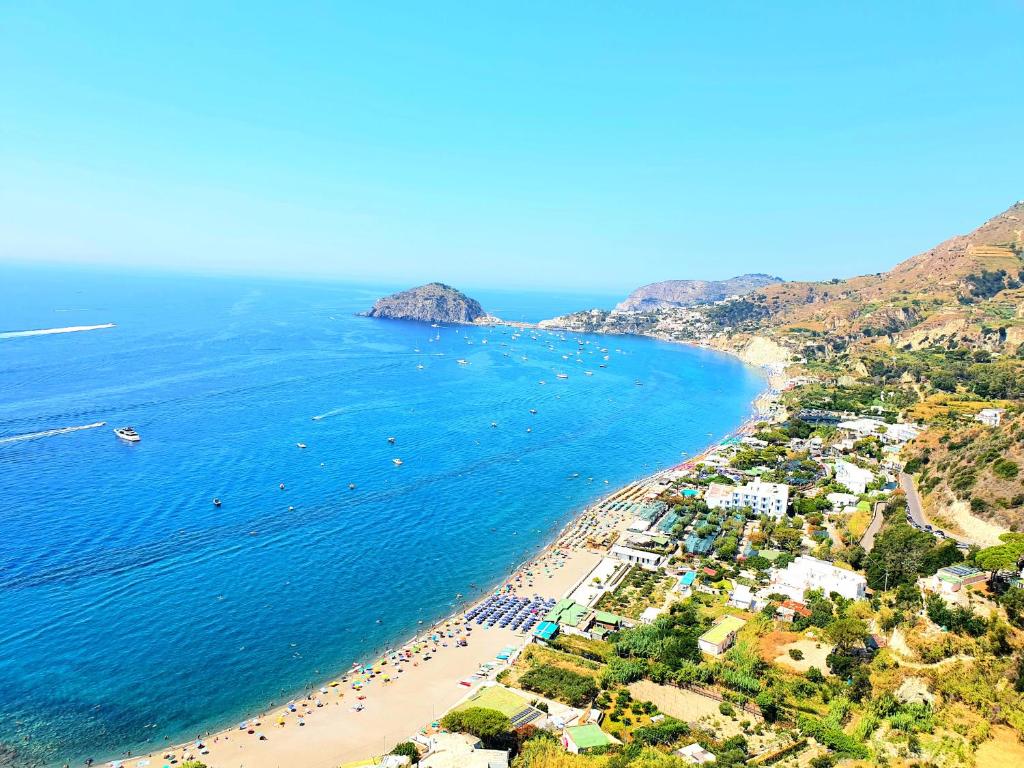The aerial view captures a stunning coastal landscape. Dominating the scene is the bright blue ocean, its crystal-clear waters seamlessly blending with the equally vivid sky, creating a continuous expanse of blue that almost merges land and sea. The left side of the image showcases a large boat, accompanied by smaller white dots that might be jet skis. On the right, a hillside covered in a mix of green vegetation and brown patches stretches downward, where it meets a sandy beige beach dotted with colorful umbrellas and people relaxing. Scattered unevenly along the hillside are various buildings connected by tiny roads. In the middle distance, a peninsula juts out into the ocean, marked by a prominent brown rock at its tip. Beachside homes are visible towards the bottom and right of the image, nestled among green grass and trees. The entire scene is bright and clear, taken during the daytime under ample natural lighting, emphasizing the outdoor beauty and the tranquility of the setting.